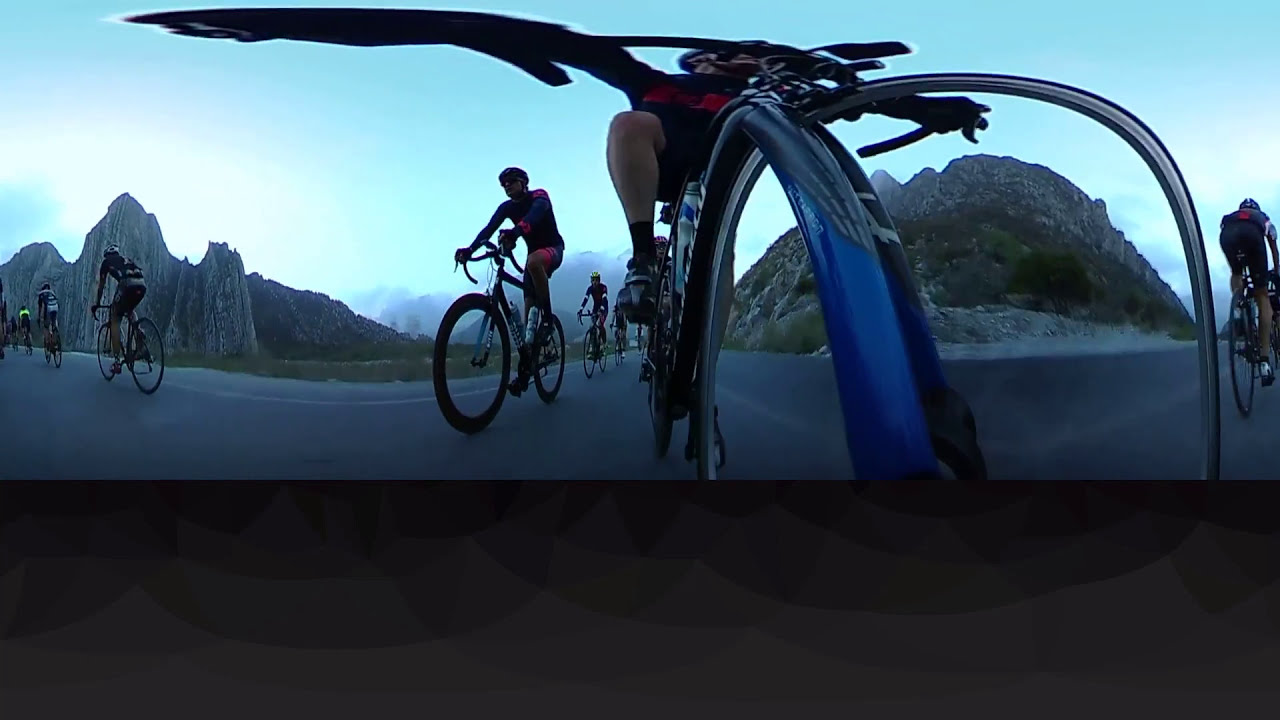The photograph captures a dynamic scene of bikers pedal biking through a striking, mountainous landscape. The image, likely taken with a fisheye lens for a panoramic effect, is shot from an unusual low angle, possibly mounted on the right side of a front bicycle fork. This unique perspective offers a semi-360-degree view, combining both front-facing and backward-facing shots. A discernible cyclist in the foreground rides a blue bike, clad in a black shirt and shorts with a horizontal red stripe, though his face is obscured by handlebars. Surrounding him are numerous bikers, anywhere from half a dozen to ten, sporting helmets and riding professional mountain bikes along a dark concrete path. The scene unfolds under a bright turquoise sky with scattered sunlight, enveloped by majestic rock formations and mountain ranges on either side, suggesting an adventurous and picturesque terrain.